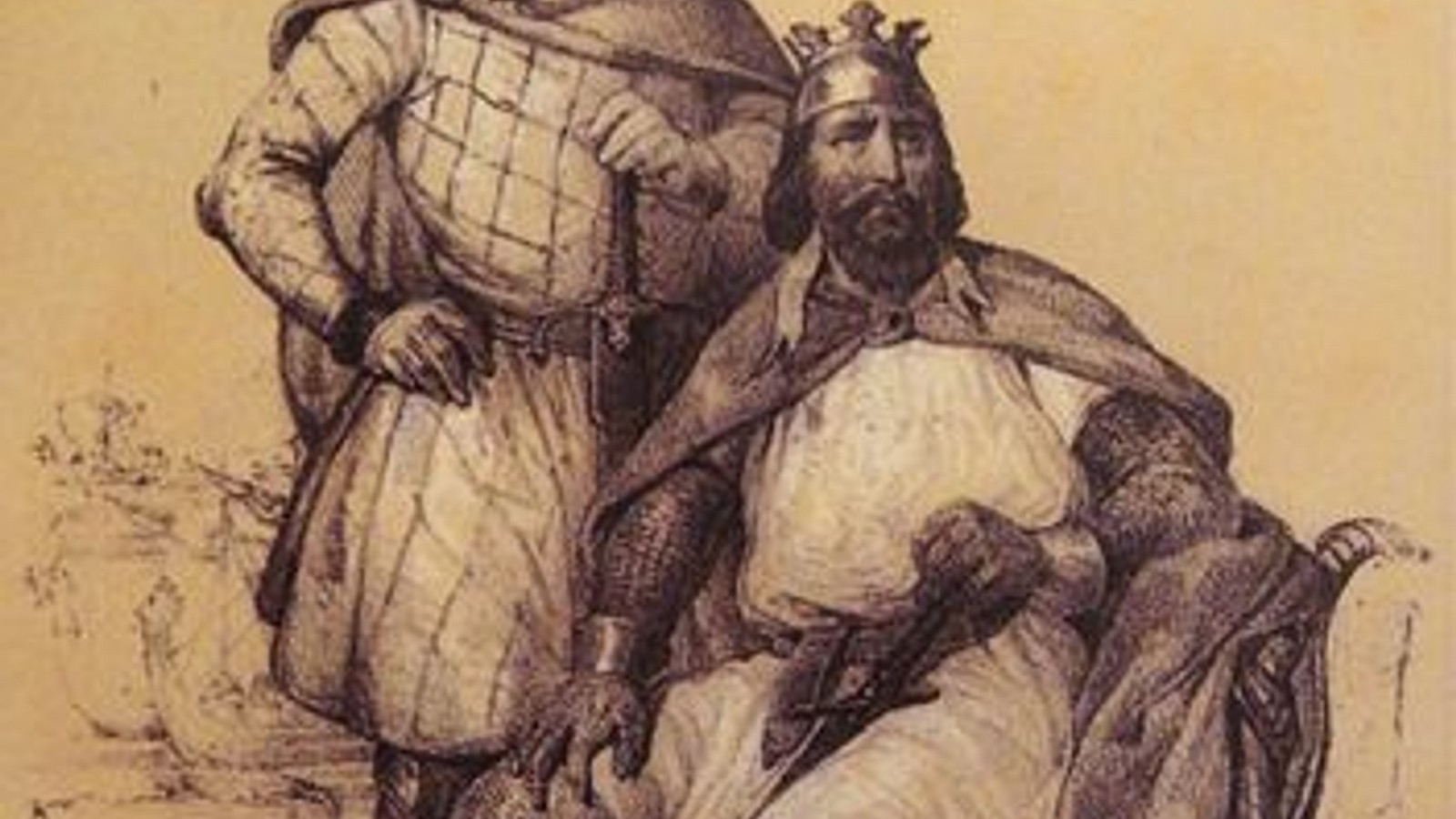The image portrays a medieval-themed artwork featuring a distinguished bearded man with long hair, sitting down. He is clad in traditional medieval clothing, including a dark cloak, a white shirt, and chainmail that covers his arms, along with metal bracelets. His left hand rests on the pommel of a sword that lies across his lap, emphasizing his readiness and status. The man also wears a crown indicating he is likely a king, and a metal belt cinches his attire. His facial features include a long pointed nose, reinforcing his distinctive appearance. 

In the background, another figure stands, partly obscured, dressed in a similar medieval cloak and armor, with a hand on his hip. The background is a beige, brownish sepia tone, giving the image an antiquated, old-fashioned print look. Sketches of Viking-style ships are faintly discernible in the backdrop, adding to the historical and epic ambiance of the scene.